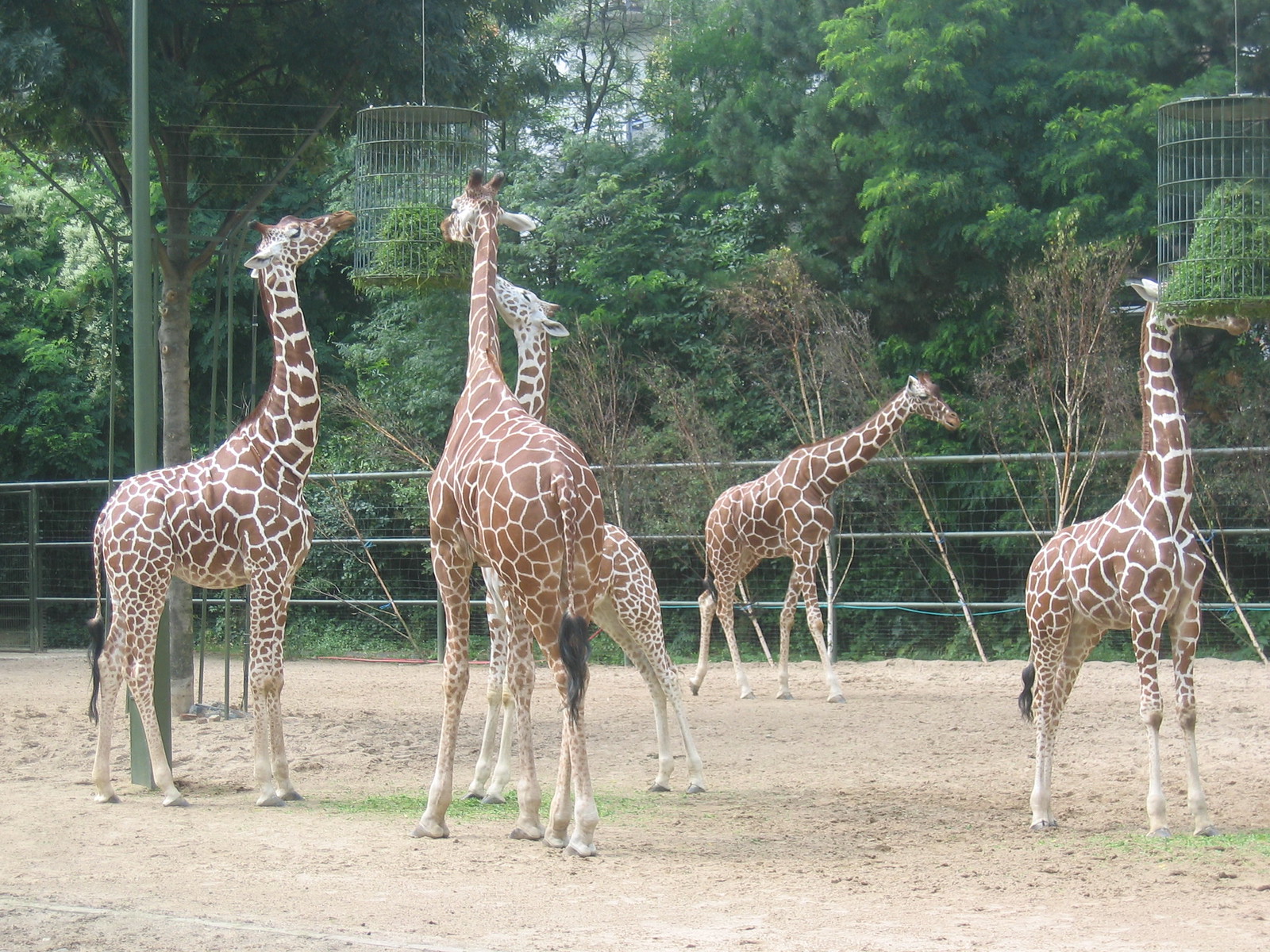In this vibrant color photograph set in a wildlife preservation, five majestic giraffes are captured in a lush environment. The backdrop is dominated by tall, green trees with a touch of blue sky peeking through at the top, providing a serene setting. At tree level, a silver fence with bluish wiring at the bottom demarcates their habitat, extending across the scene. The ground, a light gravelly beige with scattered small grass patches, stretches towards the viewer.

Central to the image, the giraffes are engaging with two hanging cages, or feeders, containing fresh green grass. On the left, a giraffe with its head fully lifted—a light and dark brown patterned beauty—strains to reach the nourishing contents. Immediately adjacent is another giraffe, seen from behind, similarly trying to feed. Just peeking above this one's back, a shorter giraffe's head is visible over the feeder's rim. Further to the right, one giraffe, slightly away from the feeding frenzy, seems to be walking with its head lowered and tail to the back. All the way to the right, another giraffe stands by a second feeder; its body angled towards the camera while its head stretches towards the left.

The detailed and dynamic positioning of the giraffes, along with their natural colors and unique spot patterns framed by the lush backdrop, highlights the serene yet lively essence of life within this preserve.